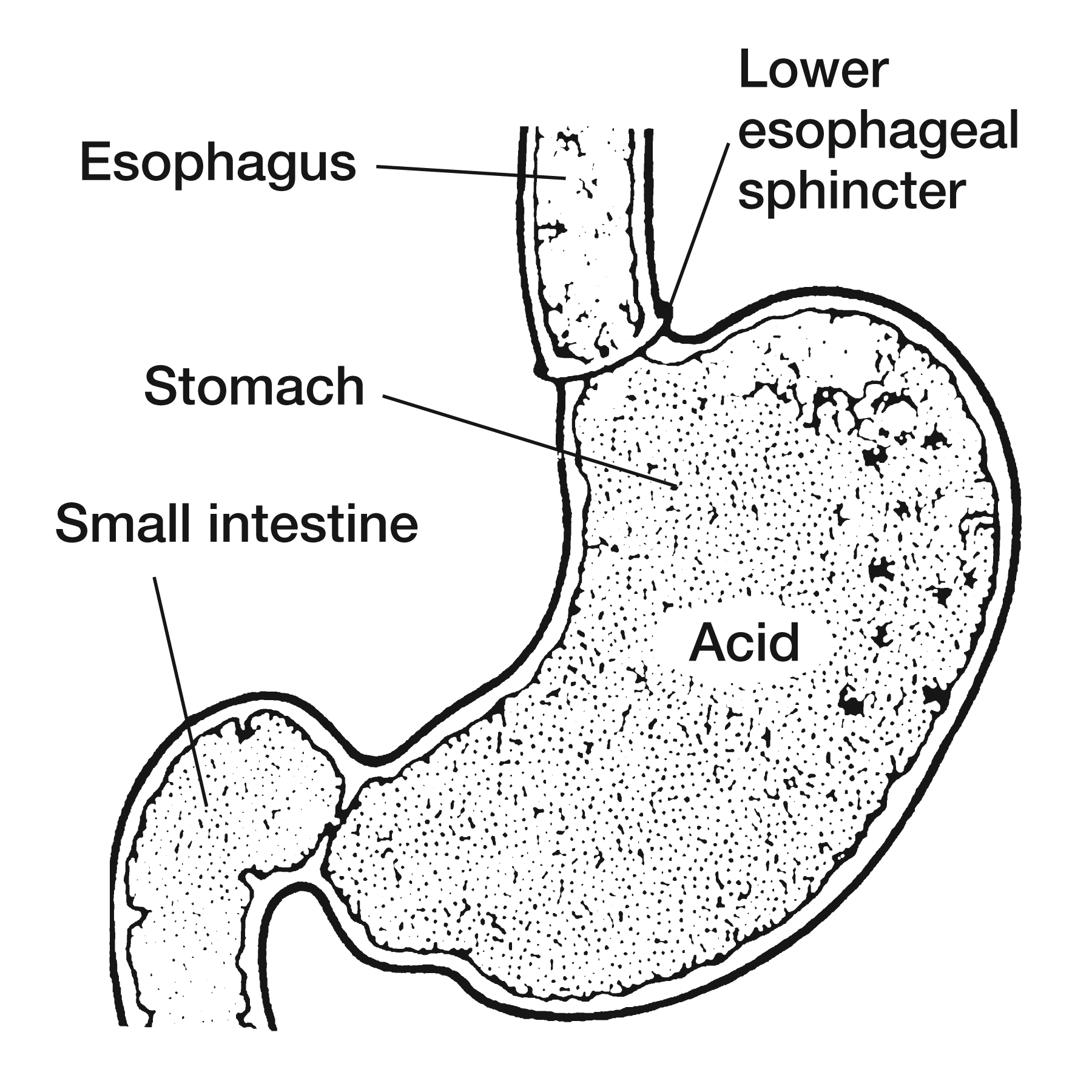This detailed, black-and-white medical illustration, likely sourced from a scientific textbook, depicts a section of the upper digestive system against a white background. The diagram prominently features the esophagus at the top, which leads down to the lower esophageal sphincter, shown as the connecting line between the esophagus and the stomach. The stomach, depicted centrally and shaped like a kidney bean, is textured with small black blotches, dots, and lines to indicate the presence of stomach acid. Inside the stomach, the word "acid" is clearly labeled. Attached to the stomach is a pipe leading downward, labeled as the small intestine, which shares similar texturing. The letters in the diagram are blocky and black, and the outlines of the organs are prominently dark with a white border beneath. The illustration is simple yet precise, clearly labeling each part without displaying the upper part of the esophagus or any sections beyond the small intestine.